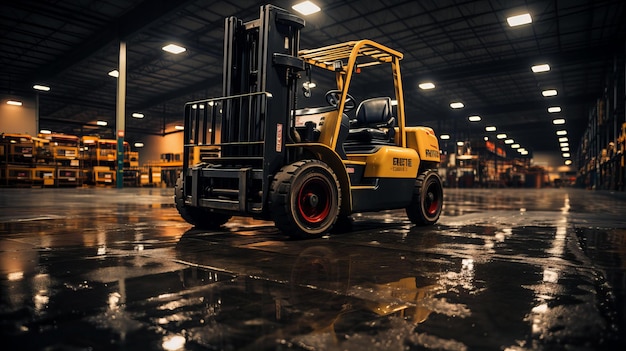This horizontally aligned, rectangular image captures a dimly lit factory or warehouse. The ceiling is lined with rows of square fluorescent lights and dotted with black poles, while skylights punctuate the metallic roof. The wet, shiny concrete floor takes up the lower half of the photo and reflects the ambient light, contributing to the dim ambiance. Dominating the center of the image is an orange forklift, its front facing left. The forklift features black tires with red rims and a protective yellow metal frame over the black seat. Though the brand name on the side is partially obscured, it begins with an 'E' in black print. The vehicle's front end, composed of black metal, is clearly visible. In the background to the left, more machinery or possibly crates, also in yellow or orange hues, are partially visible. On the right side of the image, a wide, long aisle extends further into the warehouse, bordered by shelves filled with various items. The image is taken from ground level, emphasizing the scale and depth of the warehouse space.